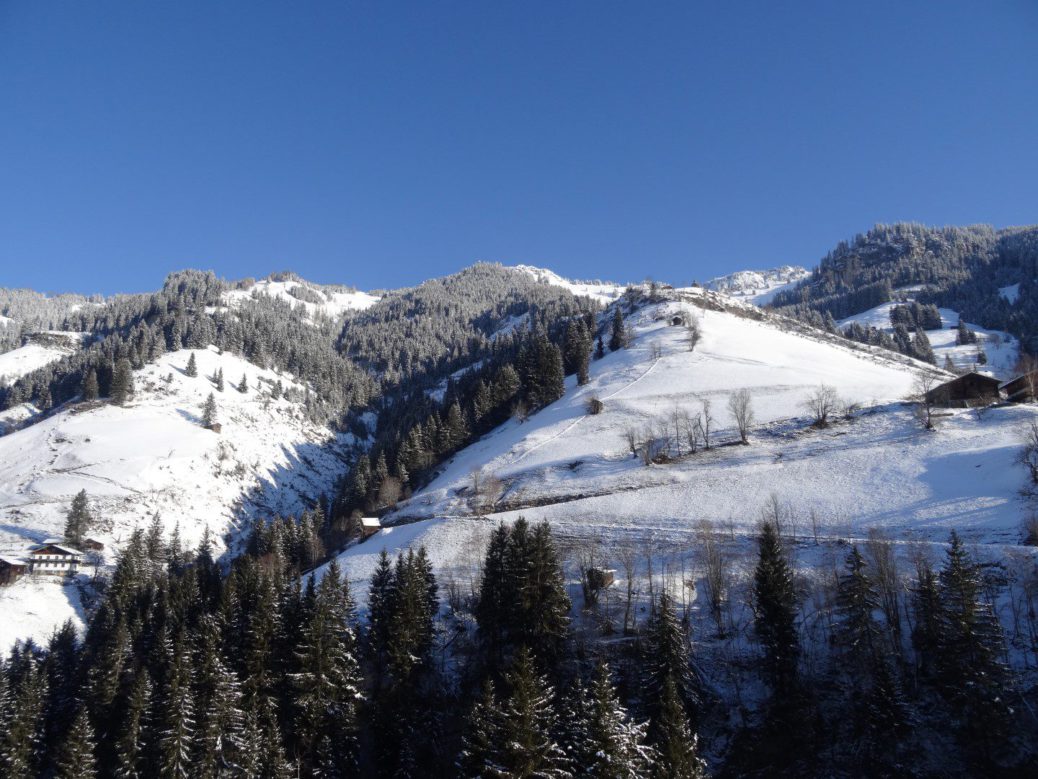The image showcases a detailed landscape of a snowy mountainside under a clear, cloudless, dark blue sky, captured during the day. The sky occupies the top 25% of the photograph, while the remaining 75% is dominated by a rugged, snow-covered mountain that slopes upward. The mountain features smooth, snowy slopes interspersed with patches where the rocky surface is visible. Pine trees, exhibiting shades of green and grey, are scattered across the mountainside, particularly dense in a large valley slightly to the left of center, and also evident in the foreground.

On the right side of the image, a large wooden lodge stands prominently, suggesting a ski resort setting. Toward the bottom left, a multi-storied building is visible, hinting at additional accommodations or facilities. A road threads its way across the landscape from right to left, connecting these structures. The predominance of blue, grey, white, brown, and off-green hues emphasizes the wintry, alpine environment.